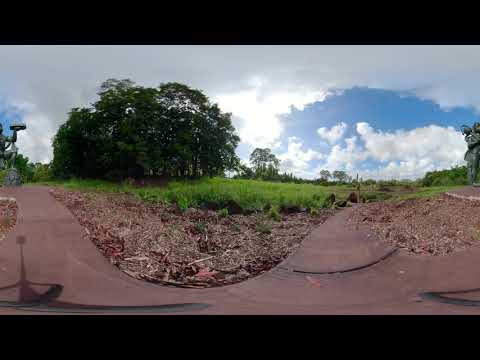The photograph captures a serene countryside pathway that presents a tranquil escape for walkers and nature enthusiasts. The pathway, paved with a reddish-brown concrete, splits into two directions—left and right—offering a choice of routes. Framing this divergence is a patch of terrain transitioning from sparse, weedy areas near the asphalt to lush green grass adorned with occasional hay, wood, and sticks further back. Prominent against the horizon is a tall, rounded tree with dark green leaves, enhancing the bucolic aura of the scene. The sky overhead is a mix of bright blue, dotted with puffy white and gray clouds that filter the sunlight, creating a soft, diffused light. Additional elements such as scattered mulch, leaves, and dead grass along the sides of the pathway further underline the natural, untamed charm of this countryside setting. The overall atmosphere conveyed is one of relaxation and leisure, making it a perfect spot for a laid-back walk or exercise session.